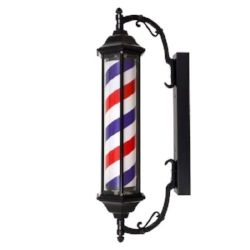The image depicts a vintage barbershop light fixture, characterized by its iconic red, white, and blue spiral stripes, indicating a place where haircuts are offered, especially for men. The cylindrical light, approximately two feet long, is positioned against a white background, devoid of any wall. The fixture is mounted on a black iron structure, presenting a flat and rectangular mounting base on the right side. This base features an intricate scroll pattern that extends outward and supports the cylindrical light with arches both at the top and bottom. The light housing consists of clear glass at the center with black caps on both ends, and three black rods running vertically—one on each side and one in the middle. These elements come together to create a universally recognized symbol of a barbershop, with its vivid red, white, and blue stripes standing out prominently against a stark white backdrop.